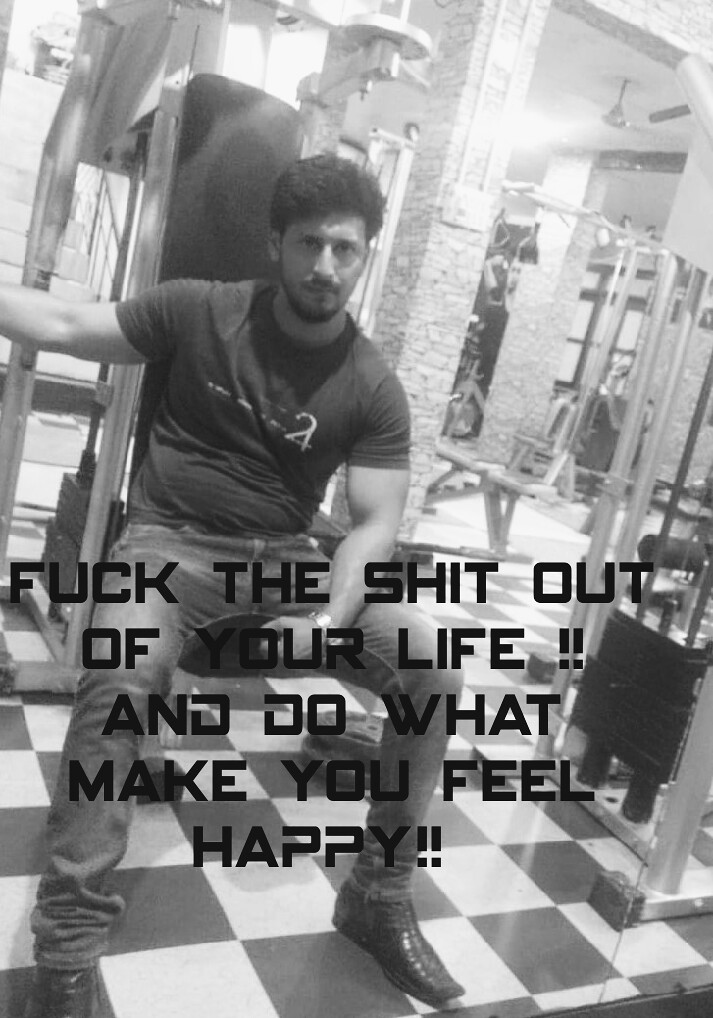The black-and-white photograph displays a man in his 30s with thick black hair and a beard, seated solemnly on gym equipment in a gym with a black-and-white checkered tile floor. His attire, a short-sleeved black shirt, jeans, and dress shoes, suggests a staged look for social media. The image, likely designed for Instagram, includes a motivational yet edgy caption: "Fuck the shit out of your life and do what makes you feel happy!" The serious expression on his face contrasts with the workout setting. Though the surrounding gym equipment is visible, the dark background adds a dramatic effect, making the man the focal point as he gazes into the camera.